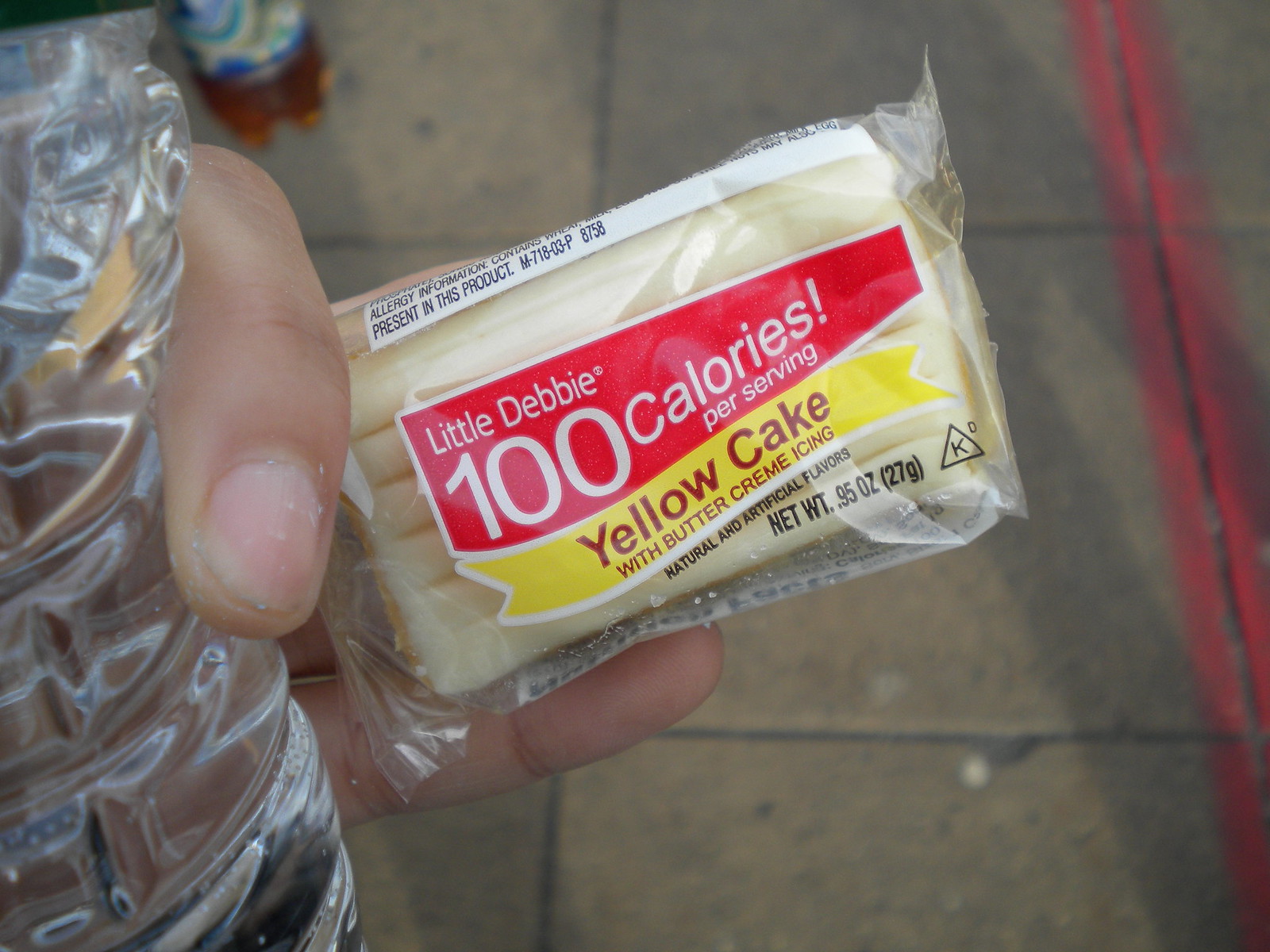In the image, an individual is holding a Little Debbie's yellow cake wrapped in clear plastic with their left hand. The packaging displays "100 calories per serving" in white text on a red banner, alongside "Yellow cake with buttercream icing" in a reddish font. The person is also grasping a clear water bottle using their thumb and index finger, while the cake is held with the remaining fingers. The background reveals an outdoor setting with a concrete sidewalk, marked by a red stripe on the right side, possibly indicating a fire lane. Additionally, another bottle is visible on the ground in the upper left corner of the image.